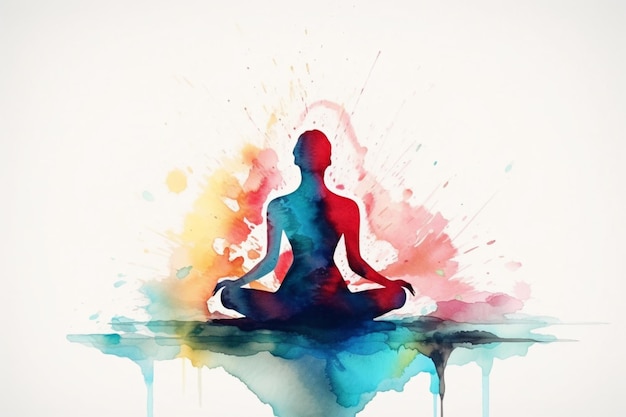This is a detailed watercolor painting depicting a woman seated in a yoga-style pose on the ground, with her legs folded so that her feet are pressing together and her knees are near the ground. Her hands rest on her knees. The artwork is characterized by the distinctive bleeding effect of watercolor, creating a dynamic and fluid appearance. The woman’s silhouette features a combination of dark blues, aquamarine, and vibrant reds, particularly in the central figure, transitioning to darker blues towards her legs. The background is a stark white with splatters and splotches of yellows, pinks, reds, and oranges that seem to radiate around her, enhancing the contrast and giving her silhouette a pronounced and almost glowing aura. Drip marks in blue and turquoise extend below her, further emphasizing the watercolor medium’s effect. Overall, the painting beautifully captures the serene yet vibrant presence of the woman in her meditative pose.